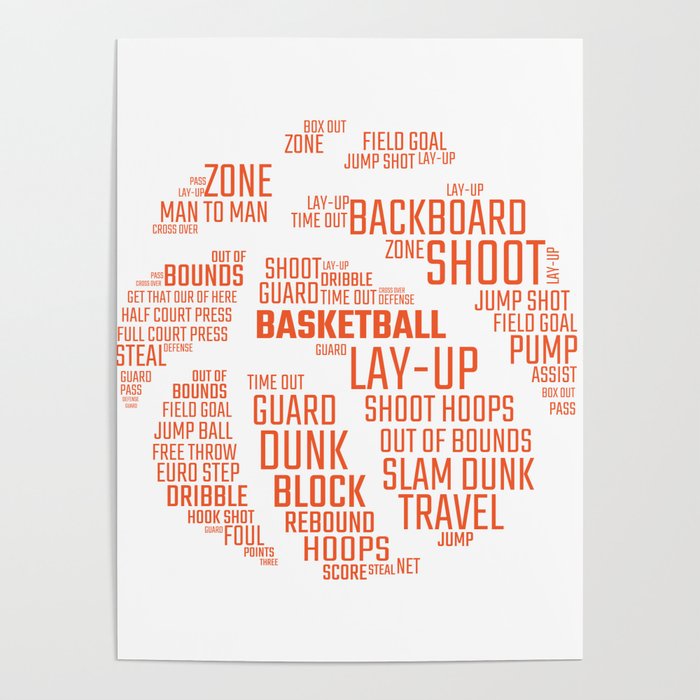This is a full-color photograph of an 8 1/2 by 11 sheet of paper with a vertically rectangular orientation, framed by a square, light blue background with a gray border that is thicker on the sides and thinner on the top and bottom. The white paper features various words associated with basketball, arranged to form the shape of a basketball. The text includes terms such as shoot, guard, dribble, timeout, basketball, layup, slam dunk, travel, jump, block, rebound, score, field goal, jump shot, and many others. These words are presented in different shades of red and orange, with some in bold and others in fainter type. The design mimics the orange sections of a basketball, with the white areas representing the lines that typically appear on a basketball. The word "BASKETBALL" is the darkest and most prominent text, located directly at the center of the composition.